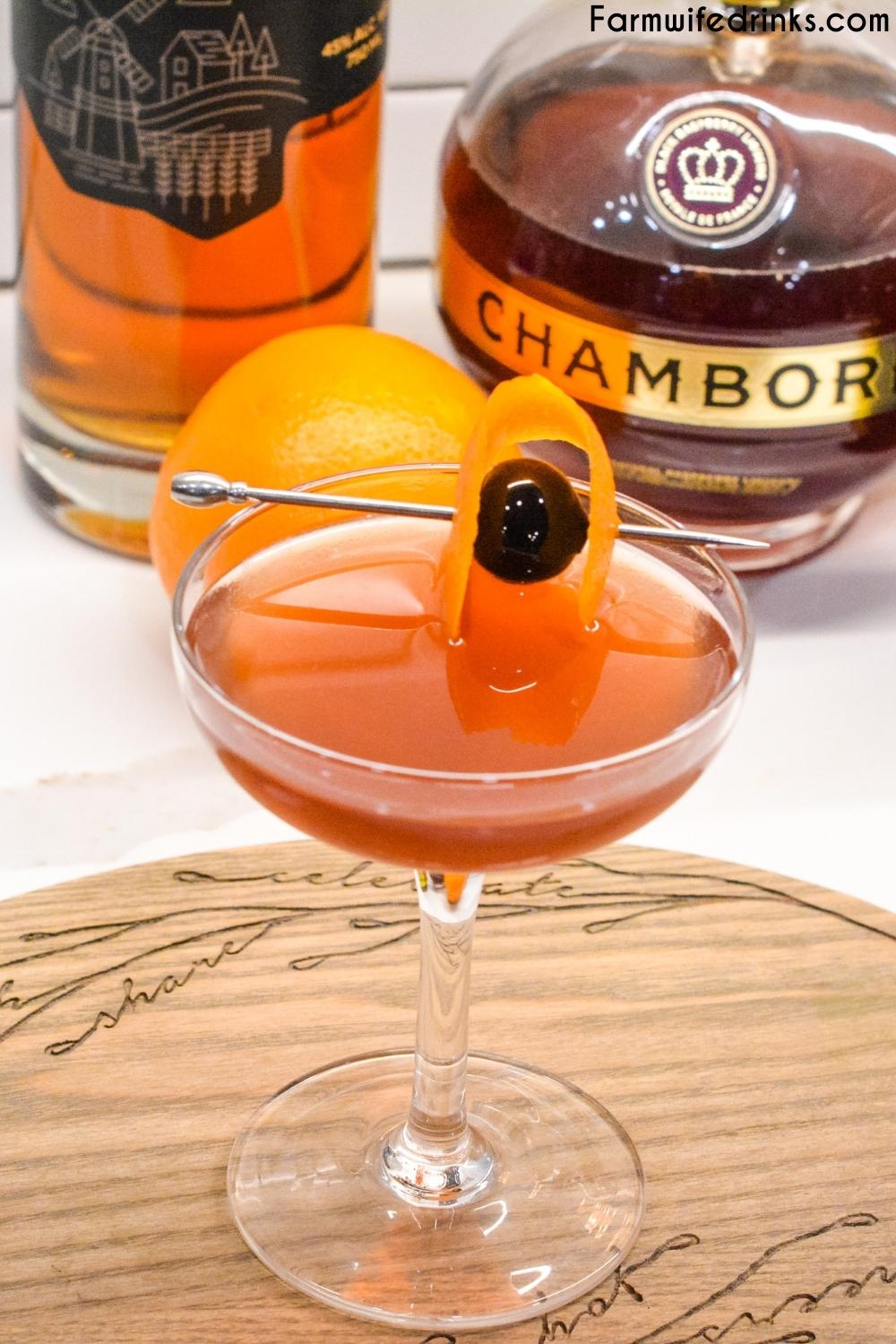The image depicts a sophisticated cocktail placed on a wooden coaster atop a white surface. The drink is served in a wide, shallow cocktail glass with a long stem and circular base. The liquid inside is a rich dark orange, almost red, giving it an inviting, syrupy appearance. Resting horizontally across the rim of the glass is a silver pin skewering a black cherry and an orange peel, with the peel dipped slightly into the drink while the cherry hovers just above it.

In the background, there is a whole orange positioned between two distinct alcohol bottles. The bottle on the left contains an amber-colored liquid and features a black label with a sketch of a farmhouse, windmill, and trees. The bottle on the right stands out due to its circular shape and deep brown liquid, adorned with a gold label that reads "CHAMBORD" and flaunts a circular logo with a crown. 

Additionally, the upper right corner of the image contains the text "farmwifedrinks.com" in black letters. The overall composition suggests a scene of refined indulgence, enriched by intricate detailing and a warm, inviting color palette.